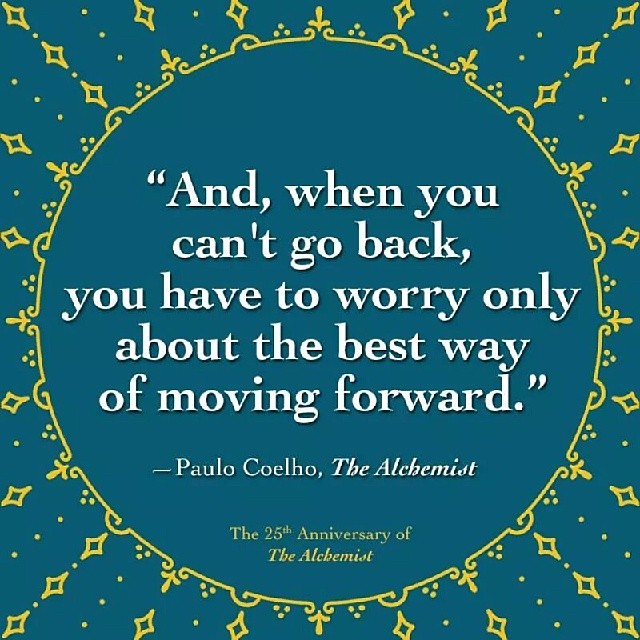The image is a square graphic with a dark blue or turquoise background, featuring a stylized circular pattern. The pattern consists of symmetrical yellow lines and four-pointed yellow stars around the edges, resembling a mandala or sun design. The center of the image, free from these patterns, showcases a quote in prominent white font that reads, "And when you can't go back, you have to worry only about the best way of moving forward." Beneath the quote, in smaller yellow font, it states, "Paolo Coelho, The Alchemist". Further down, also in yellow, it mentions, "The 25th anniversary of The Alchemist." The image is visually balanced with its intricate yellow designs and contrasting text, giving it a celebratory and inspiring feel.